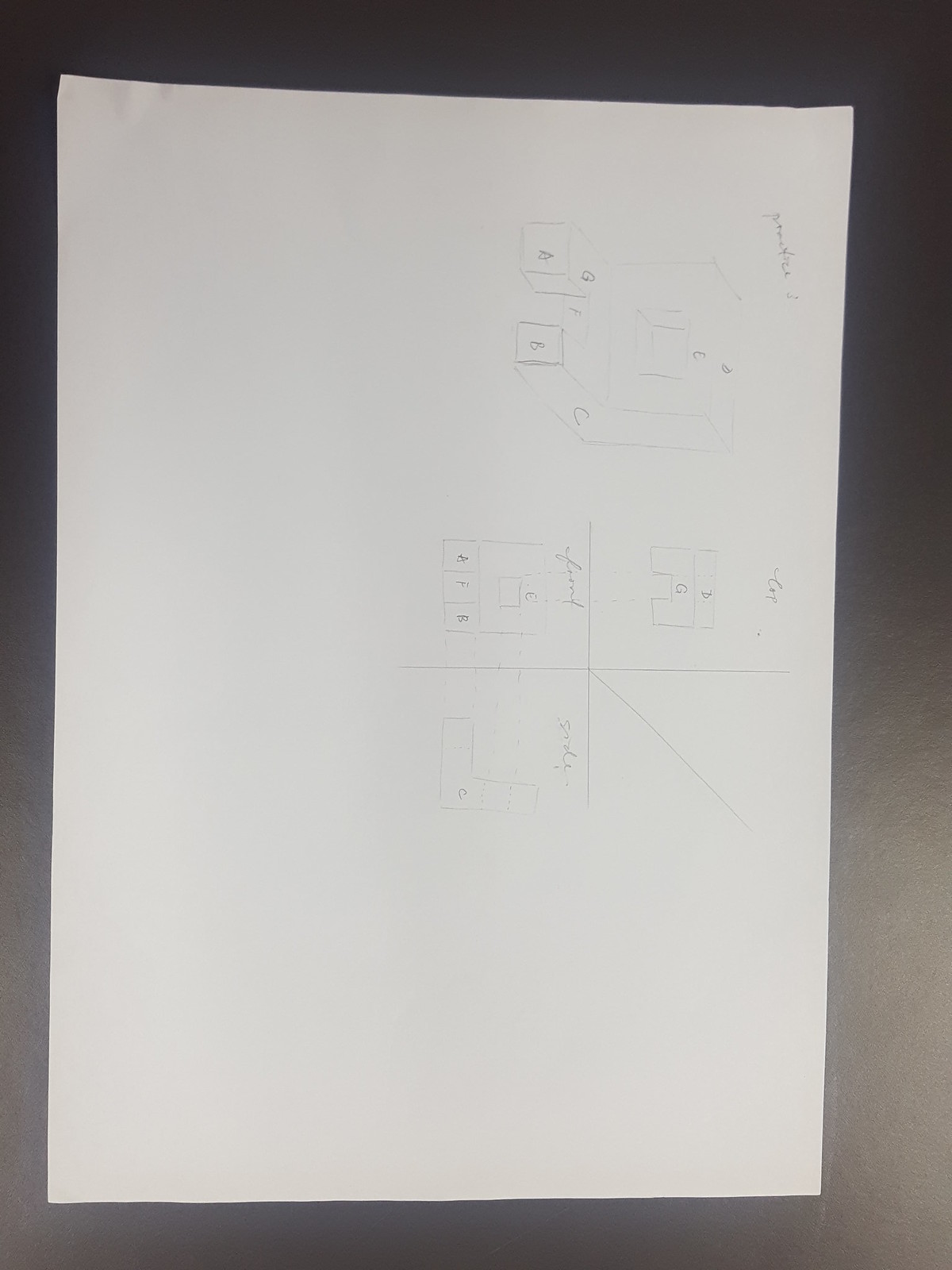The image features a background that transitions from dark at the top to lighter shades towards the bottom, likely due to the flash of a camera or an external light source. Positioned towards the left side of the image, there is a rectangular piece of paper oriented horizontally. This paper showcases primitive pencil sketches, including various square boxes and simple shapes. Notably, near what would be the upper left side of the paper, there's a written cursive inscription that is difficult to decipher. Closer to the center of the paper, the word "cop" appears to be written in cursive. The paper is further adorned with four square boxes, lines, and simple geometric shapes, some of which are labeled with letters: A, B, C, D, E, D, and G. The intent or meaning of these labels is unclear based on the image alone.